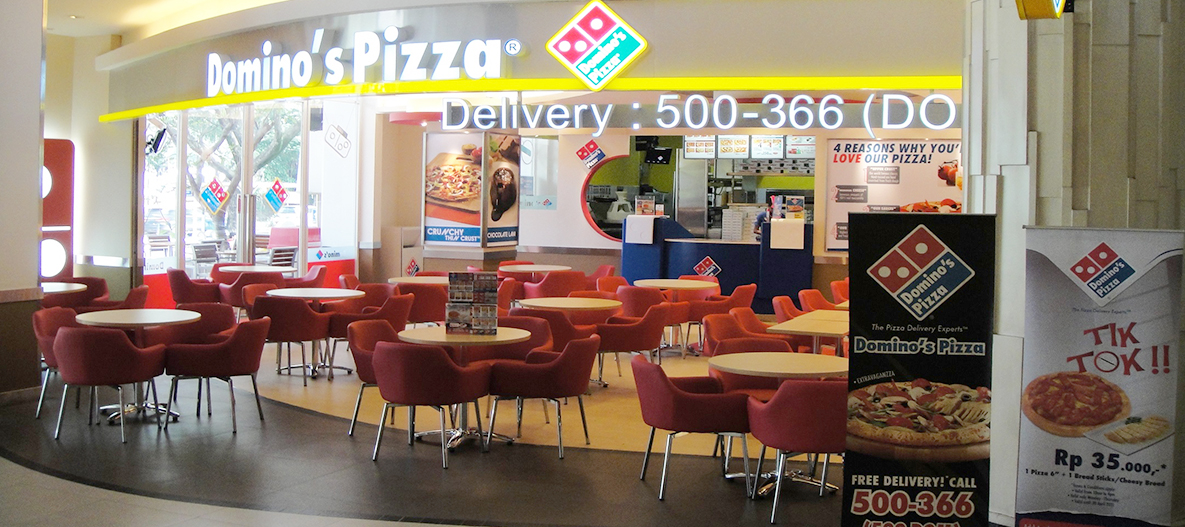Inside a Domino's Pizza restaurant, the scene is empty, revealing an array of round tables with matching red chairs, all featuring chrome-colored legs. The tables are set against a partially beige and partially black floor. In the right bottom corner, there are prominent signs, one of which is a slightly tilted black square stating "Domino's Pizza", "Free Delivery 500-366", and a pizza image. Adjacent to it is a white sign with "TikTok", an image of a pizza, and "RP 35.000". In the background, illuminated white letters at the top proclaim "Domino's Pizza", with a yellow line running underneath across the room. Below this, a counter with blue stands sits in front of menu windows where people place orders. Additional wall posters featuring pizzas and promotional messages adorn the space. Outside the entrance, visible through the windows, stands a tree with green leaves.